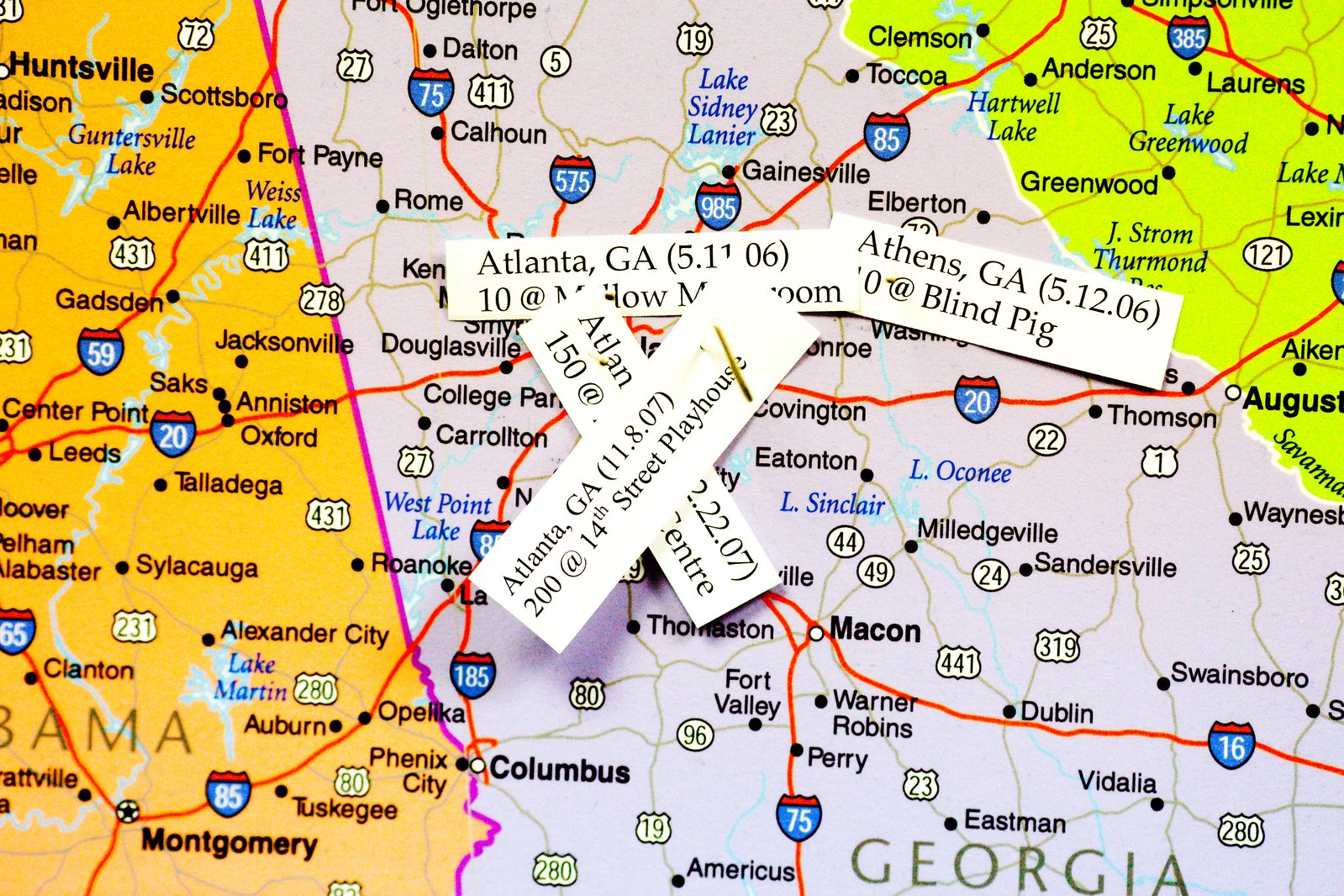This image is a close-up of a horizontal and rectangular map, primarily showcasing the state of Georgia, which is colored in light purple. The map includes neighboring states: Alabama to the left with an orange background, and South Carolina to the right, which shifts to a green color. The map features numerous red and gray lines representing highways and roads, with blue shields indicating interstate numbers such as 59, 20, 85, 65, 75, 575, 985, 16, and 385.

Notably, the map contains four white rectangular cutouts with specific addresses typed on them. These cutouts are horizontally aligned and include details such as: 
1. "Atlanta, Georgia, 51106"
2. "Atlanta, Georgia, 11807, 14th Street Playhouse"
3. "Atlanta, and the rest is obscured"
4. "Athens, Georgia, 51206, Blind Pig"

Additionally, in the lower right corner, prominently labeled in big letters, it reads "Georgia." This map not only highlights key interstates but also provides detailed locational address tags, enhancing its informational depth.